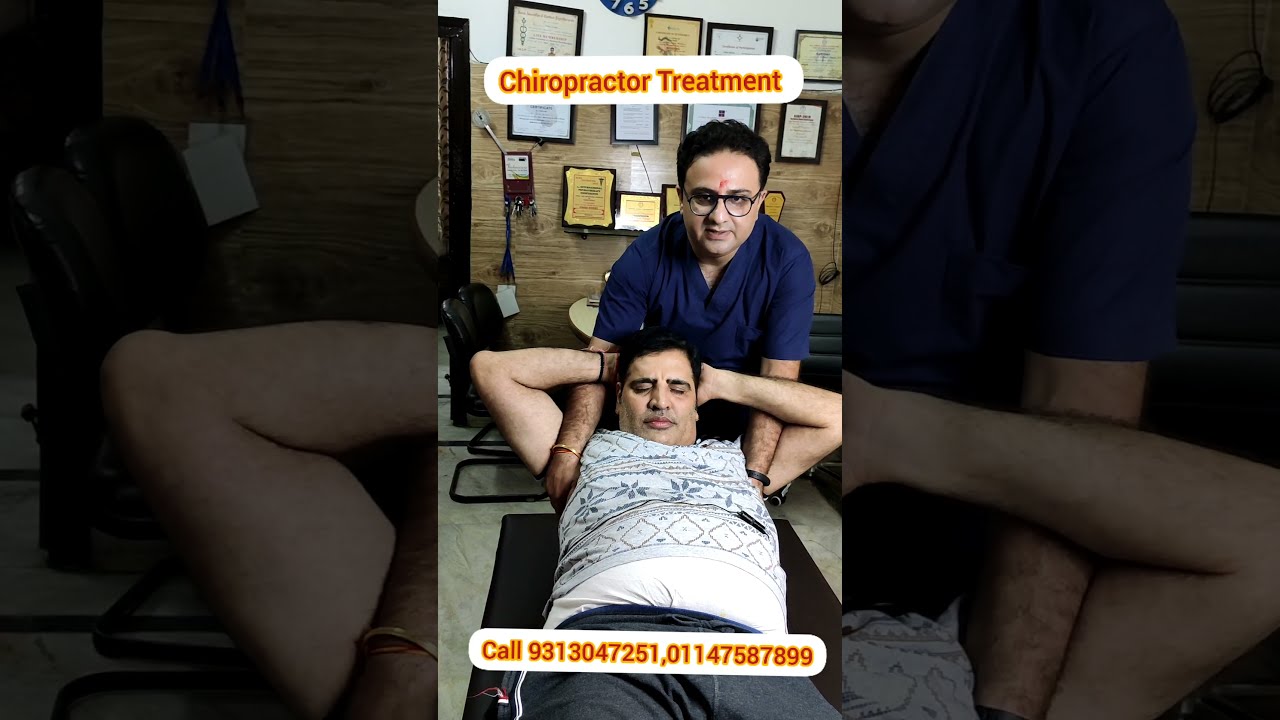The image is composed of three panels, with the central panel serving as the main focal point and the left and right panels displaying darkened, enlarged versions of it. The central panel prominently features a photograph of a chiropractic treatment session taking place in a well-decorated office. The office walls are adorned with numerous framed diplomas and certificates, organized in three rows: four in the top row, four in the middle, and at least five in the bottom row. The room also features a black chair, a brown table, and another black chair situated on the right side.

In the photograph, two Middle Eastern men are present. The chiropractor, dressed in a dark blue scrub top, wears black-rimmed glasses and a red painted dot on his forehead. He also has short black hair and is wearing a watch and a bracelet. He is in the process of administering an adjustment to a second man who is lying on a black table. The patient is clad in a white patterned shirt and gray pants, with his arms positioned behind his head. 

Text is displayed both at the top and bottom of the central panel. At the top, it reads "Chiropractic Treatment," while at the bottom, two phone numbers are provided in red font: "Call 931-304-7251, 011-4758-7899."